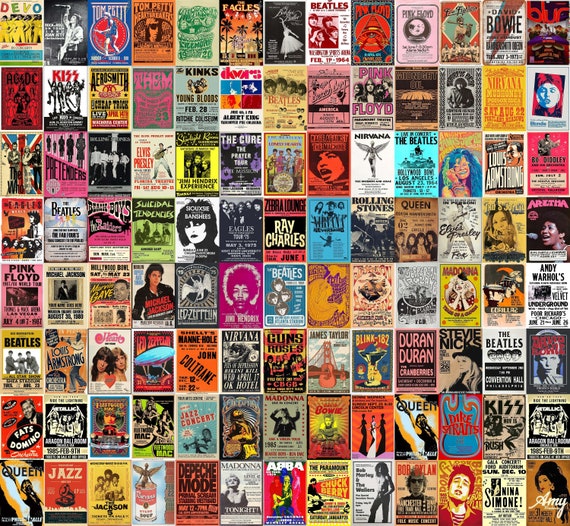This image showcases a vibrant and colorful collage of 104 album covers and band posters, arranged in a grid with 13 columns and 8 rows, creating a squarish overall appearance. Each individual poster or album cover features striking graphics and prominently displays the title of the artist. The collection spans various genres, including rock and roll, jazz, older music, and heavy metal. Notable artists and bands featured include Queen with Freddie Mercury, Michael Jackson, Nirvana, Madonna, Kiss, Rick Charles, Pink Floyd, Devo, The Beatles, and David Bowie. The diverse, multi-colored graphics on each piece contribute to a visually stimulating mosaic that resembles a spread of Skittles.